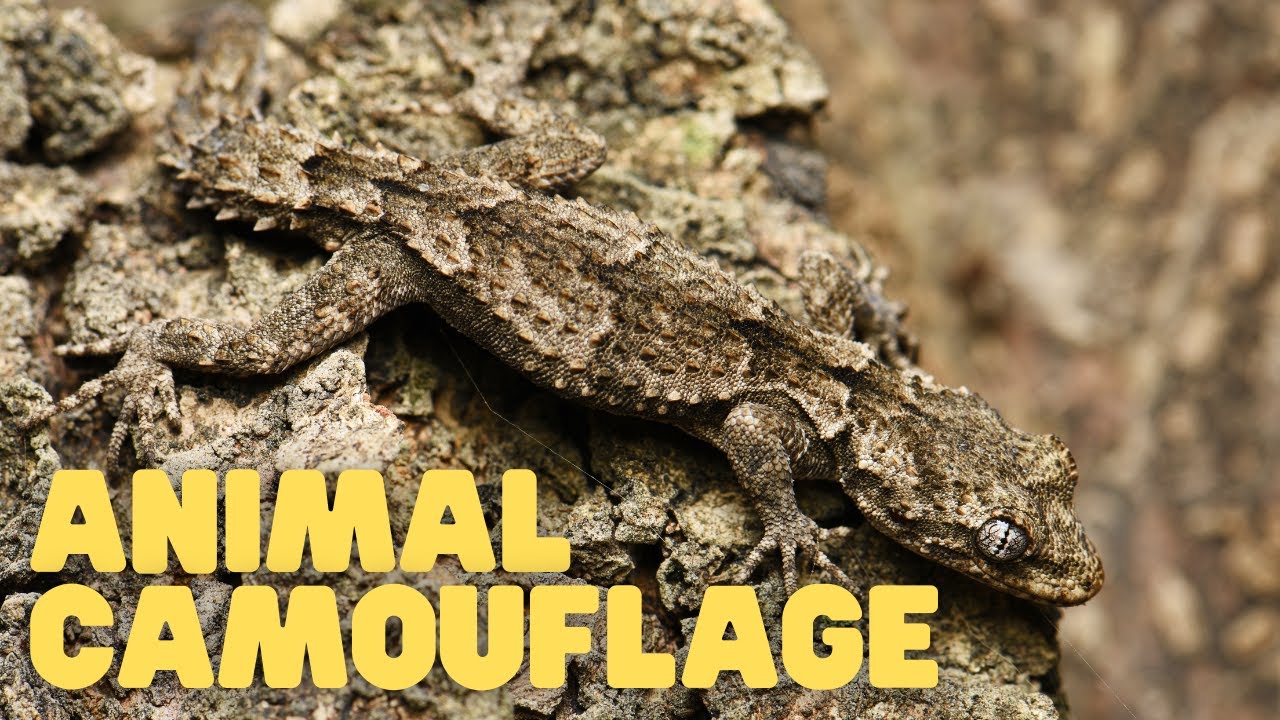In this outdoor photograph, a camouflaged gecko or lizard is nearly indistinguishable from its surroundings. Positioned on a rough, brownish rock, this small reptile exhibits remarkable camouflage, its skin mimicking the rock's texture and colors perfectly. The lizard has a mix of brown, tan, green, and gray hues, with scaly skin and spikes on its tail. It's so well-blended into its environment that it’s almost invisible unless you look closely. Its eyes are closed, further helping it melt into the background. The image prominently features the text "ANIMAL CAMOUFLAGE" in bold yellow letters at the bottom left, emphasizing the creature's impressive natural disguise.